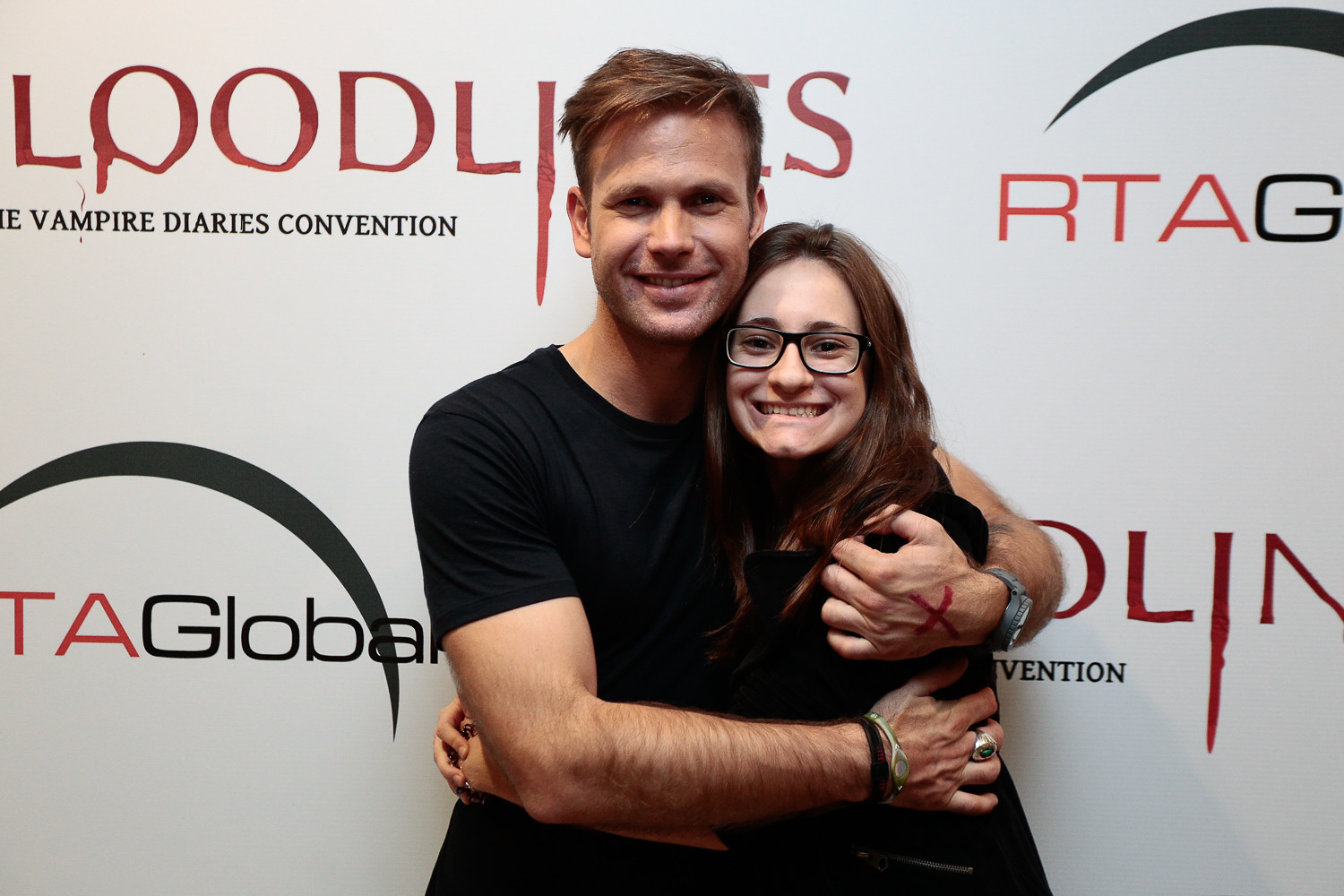This full-color indoor photograph captures a joyous moment at the Vampire Diaries Convention. In the image, a man and a woman are closely embracing, both of them smiling brightly. The woman, who is wearing glasses, has her arms wrapped affectionately around the man, while he reciprocates the gesture. The man is notable for his detailed accessories, including a ring on his right middle finger, multiple wristbands, a watch on his left wrist, and a red 'X' marked on his left hand. He is dressed casually in a black short-sleeved t-shirt. They stand against a backdrop featuring the logo "RTA Global" and partially obscured signage referring to "Bloodlines," which relates to the Vampire Diaries Convention, hinting at a cosplay event possibly involving actors from the show. The overall ambiance resembles a red carpet event with various sponsor names visible in the background.